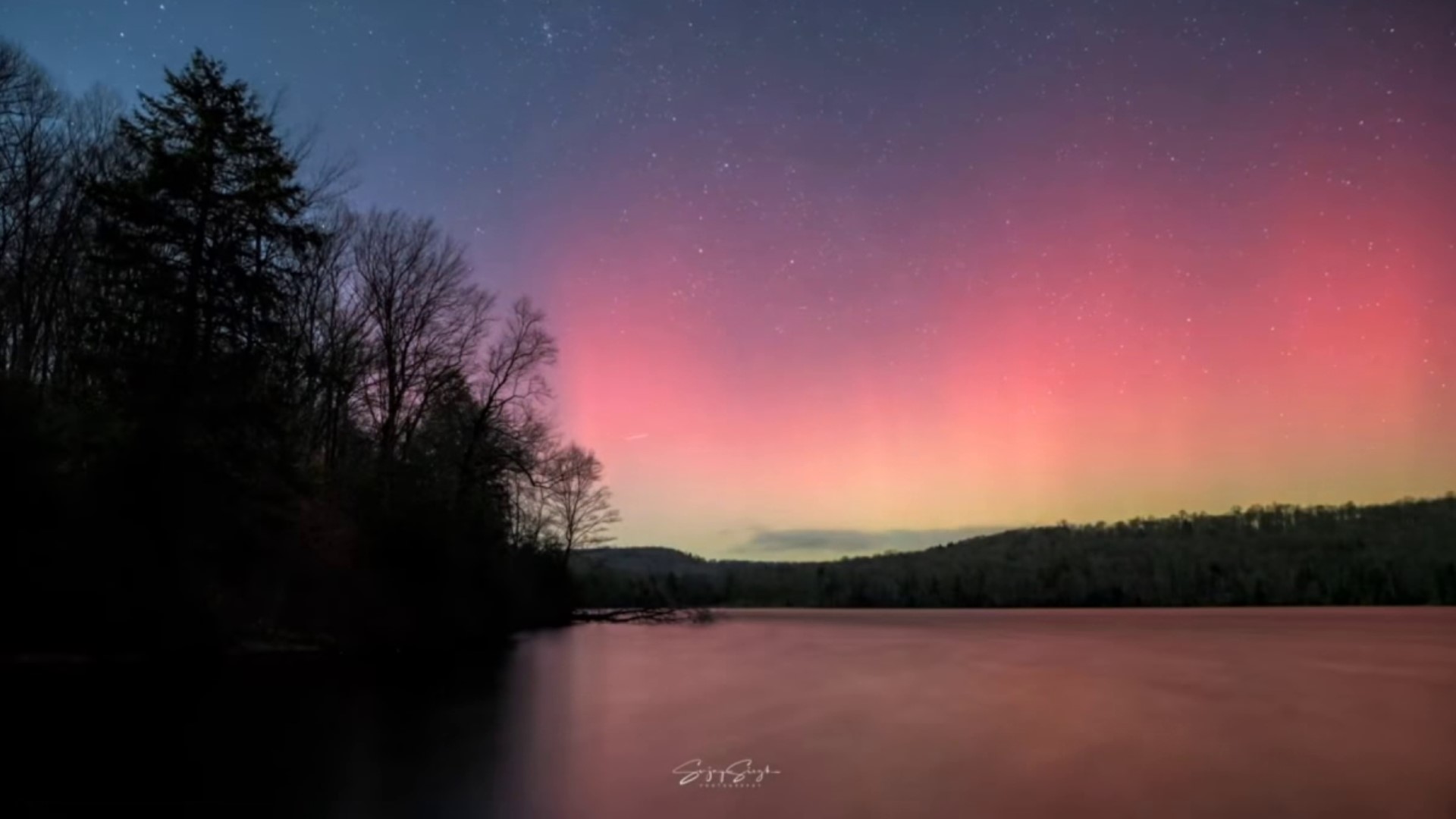This is a highly detailed image, likely a painting, capturing a serene sunset over a calm lake enveloped in tranquility. The water is perfectly still, creating a mirror-like surface that reflects the soft, enchanting colors of the sky. To the left of the scene, tall, overhanging trees provide a dark silhouette against the ethereal backdrop, adding depth to the composition. 

The sky is a spectacular blend of pinks, greens, and yellows, reminiscent of the Aurora Borealis, transitioning seamlessly into a bluish-purple hue towards the top. Faint starlight punctuates the night sky, heightening the peaceful ambiance. Additional hills are visible in the far distance on the right side of the lake, contributing to the overall depth and balance of the scene.

Occupying the bottom center of the image is some cursive script, albeit indecipherable, adding a touch of mystery and elegance, enhancing the 'postcard-perfect' quality of this landscape. The entire composition radiates softness and serenity, making it a quintessential depiction of natural beauty at twilight.